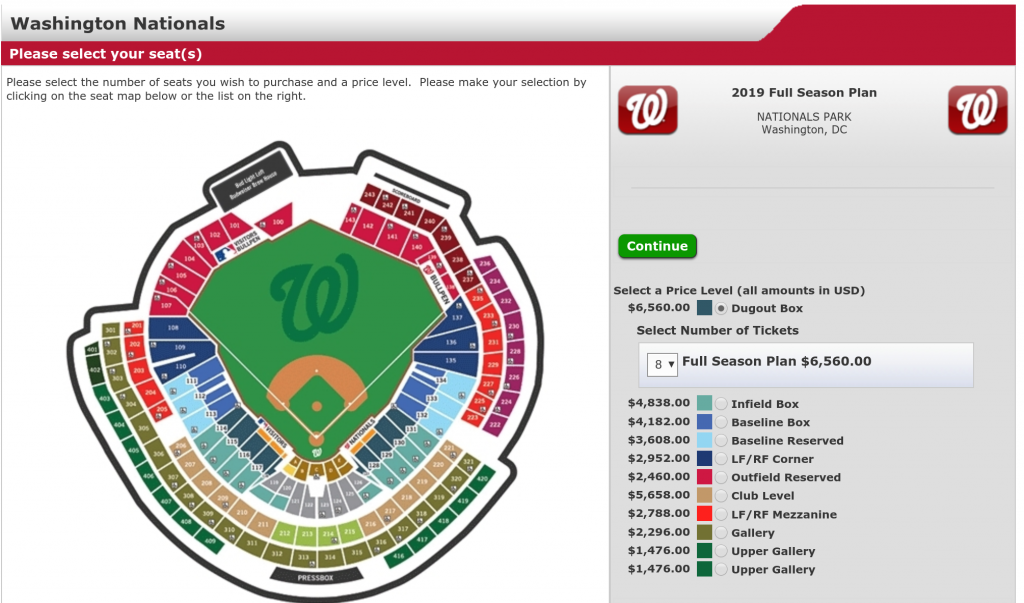The image showcases the Washington Nationals ticket purchasing page on their website. In the upper left-hand corner, "Washington Nationals" is prominently displayed in black text against a gray background. Below this, a red tab resembling a file folder extends down. Within this red tab is an option labeled “Select Your Seats” in white text.

Beneath the navigation bar, there is a detailed schematic of Nationals Park, allowing users to see all available ticket options for different sections of the stadium. A prompt instructs users to select the number of seats and price level they wish to purchase, with choices available through an interactive seat map or a list positioned to the right side of the page.

Further down, the page details ticket plans, such as the "Washington Nationals 2019 Full Season Plan" for Nationals Park in Washington, DC. Users are prompted to continue by clicking a green button labeled “Continue.” Price levels are clearly marked, with all amounts displayed in US dollars. For instance, a Dugout Box would cost $6,560, and the user depicted in the image has opted to purchase eight of these premium tickets, possibly indicating a significant expenditure either personally or on behalf of a company. The cheapest season ticket option is listed at $1,476 for the Upper Gallery.

The page is user-friendly and meticulously designed to facilitate the selection and purchase of season tickets, offering a range of pricing to suit different budgets.